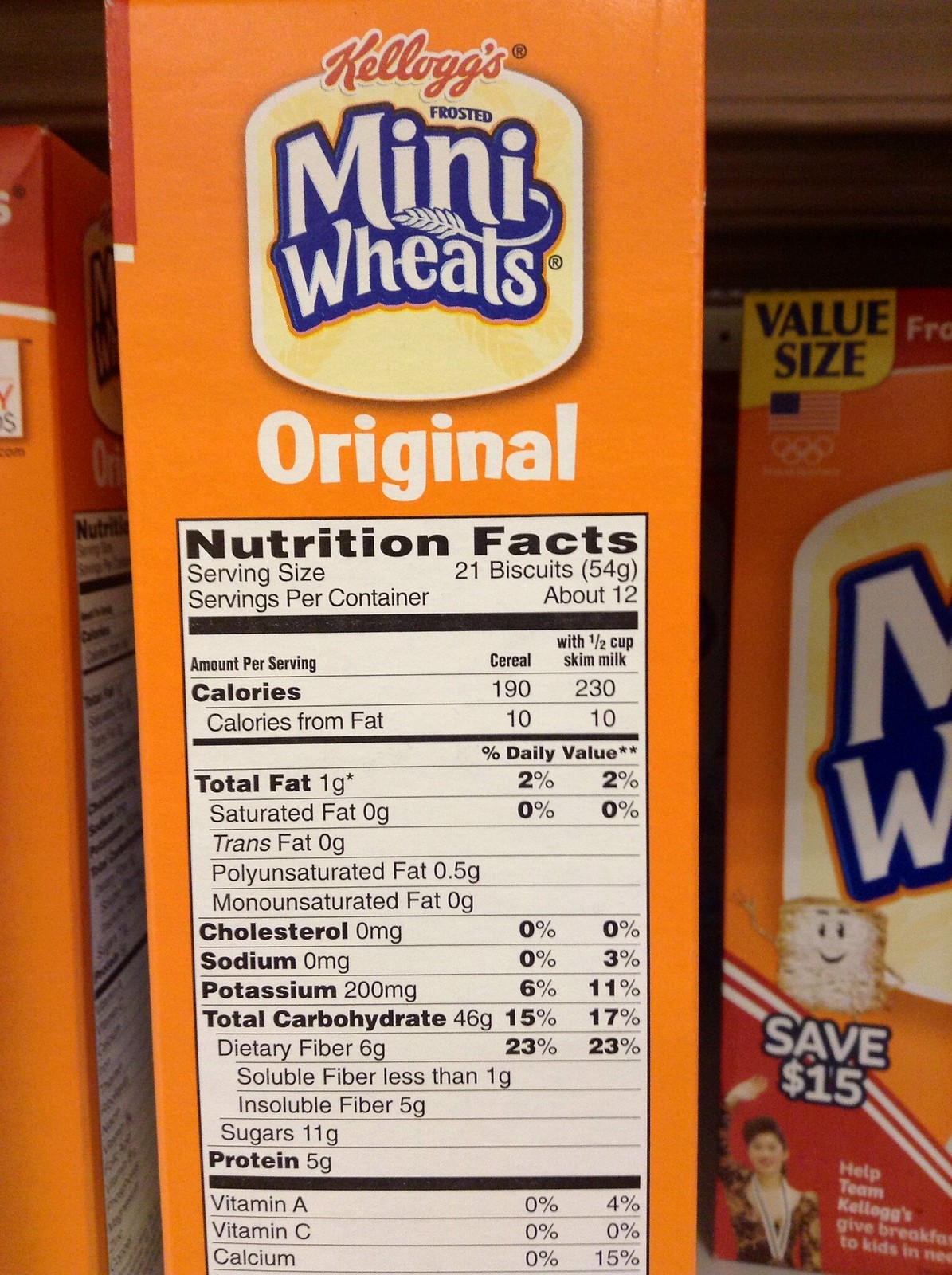The image features the side panel of an orange box of Kellogg's Frosted Mini-Wheats cereal, prominently displaying nutritional facts. The top portion of the image shows the underside of a grocery store shelf, and adjacent boxes of similar cereal can be seen on both sides. The panel includes a yellow rounded square with "Mini Wheats" in white text outlined in blue, and "Kellogg's" in red lettering at the top. Above "Mini Wheats," it specifies "frosted" in small blue font. Just below, "original" is written in white text. The nutritional information lists a serving size of 21 biscuits (54 grams) with approximately 12 servings per container. Each serving without milk provides 190 calories, 1 gram of fat (2% of daily value), 0 mg of cholesterol and sodium, 200 mg of potassium (6% daily), 46 grams of total carbohydrates (15% daily), 6 grams of dietary fiber (23% daily), 11 grams of sugar, and 5 grams of protein. The panel also details changes when consumed with milk, altering the calories to 230 and adjusting values for potassium (11%), total carbohydrates (17%), dietary fiber (also at 23%), as well as providing 4% of your daily calcium needs. Additionally, an orange box with a red corner shows an Olympic athlete and the message "Help Team Kellogg's give breakfast to kids," along with a "Save $15" promotion.